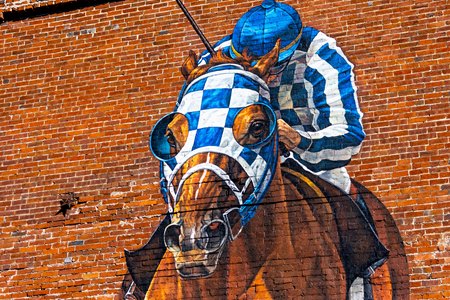This photograph captures a striking mural painted on an aged red brick wall, characterized by various shades of red and orange and visible signs of wear and tear. The mural itself is highly detailed and realistic, creating an almost three-dimensional effect as if the horse and jockey are bursting out of the wall towards the viewer. The scene features a dynamic racehorse and its jockey in mid-race. The horse is a beautifully rendered reddish-brown with a blue and white checkered head covering, complete with eye openings, enhancing its lifelike appearance. The jockey, whose face is obscured by his downward gaze, is dressed in a matching blue and white checkered uniform with striped sleeves and a blue cap. He grips a riding crop in his right hand, adding to the sense of motion and urgency. The level of detail, from the horse's musculature to the intricate patterns on the jockey's attire, makes the mural incredibly vivid and almost tangible against the textured backdrop of the brick wall.